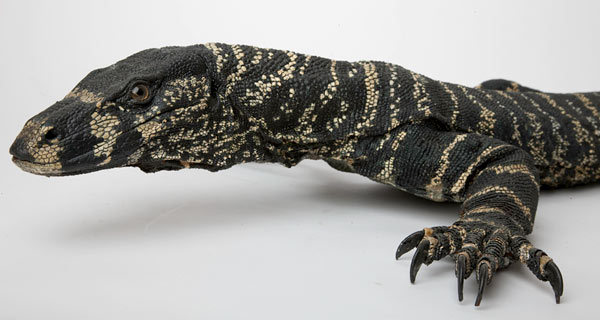The image captures the front half of a large, black lizard, possibly a savannah monitor or Komodo dragon, resting on a white surface. The lizard's skin is covered in rough, scaly textures with intricate patterns formed by white dots and tan striping. It possesses a lanky, elongated body and a prominently flat, elongated head with a distinctive brown eye. The creature's left front leg is visible, showcasing five long, curvy, sharp black claws. Overall, the lizard appears very dry and scaly, and its head is slightly lifted off the ground, presenting a detailed view of its rugged and majestic appearance.